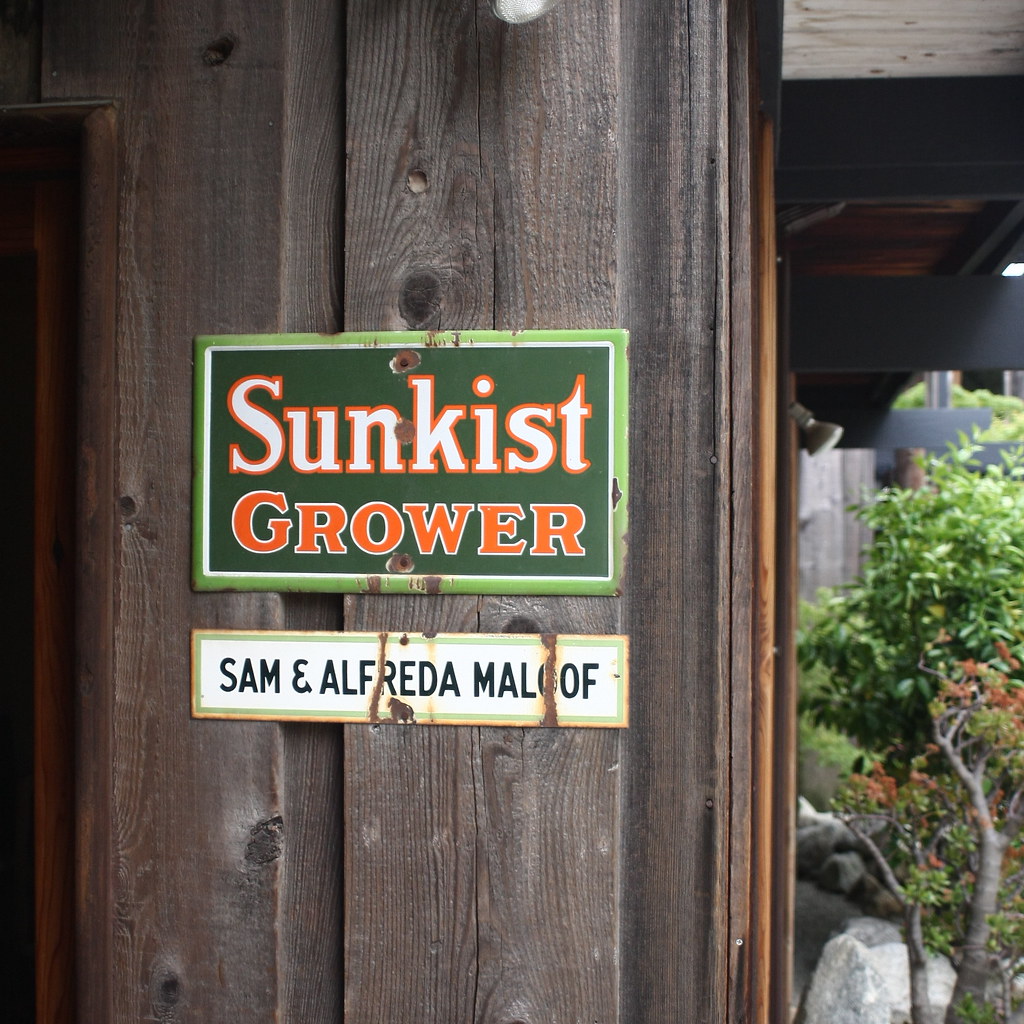The photo showcases two vintage, weathered signs mounted on a vertical wooden fence that is dark brown to blackish in tone. The upper sign is predominantly dark green with a light green border inside a white outline. It features the words "Sunskist Grower," with "Sunskist" in white text outlined in orange, and "Grower" in orange text outlined in white. Below it hangs a smaller, rusted sign with a white background and green border, which reads "Sam and Alfreda Maloof" in black text, though rust obscures parts of the letters "O" in "Maloof" and "R" in "Alfreda." To the right, the fence has an open doorway revealing a garden area with trees, rocks, grass, and a floodlight attached to the side of a structure. A green bush and a wooden fence can also be seen in the background, contributing to the rustic, outdoor ambiance.